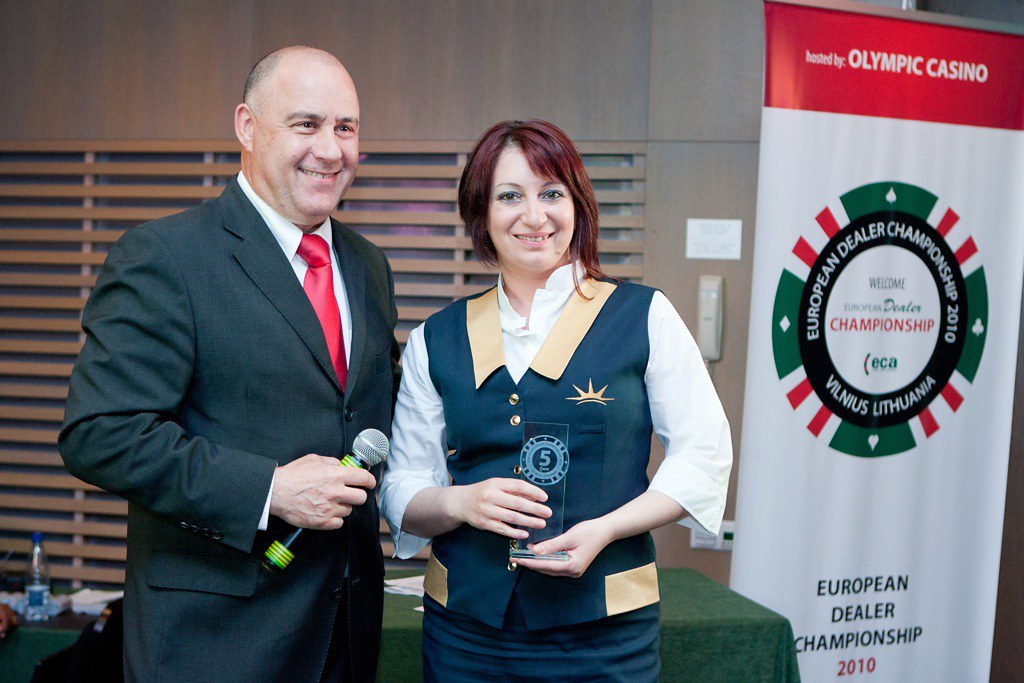In this indoor image, we see a man and a woman standing centrally. The man, who is bald and slightly older, is wearing a dark gray suit with a red tie and a white button-up shirt. He is smiling and holding a microphone in his right hand. Beside him, on the right, is a woman with dyed red hair, styled short on one side and long on the other. She is of Caucasian descent and is wearing a white button-down shirt under a blue sleeveless vest with a tan collar and gold buttons, displaying a crown logo on the chest. She holds a small glass trophy featuring the number 5 inside a poker chip design.

Behind them is a brown wooden wall with a window featuring horizontal slats. A rectangular table covered with a green cloth, which holds some papers and a bottle of water, is positioned behind the speakers. To the right of the speakers is a large banner that occupies about a quarter of the image. The banner has a red header with white bold print reading "Hosted by Olympic Casino." Below, in the center of the banner, is a white circle outlined in black with red, white, and green stripes inside. The text inside the circle reads, “Welcome European Dealer Championship” in varying colors: “Welcome” in black, "European Dealer" in green, and "Championship" in red. The black ring around the circle reads "European Dealer Championship 2010 Vilnius, Lithuania" in white. At the bottom of the banner, “European Dealer Championship” is written in green, with "2010" in red. The room's color scheme includes tan, brown, red, white, green, dark blue, and gray, emphasizing the professional and competitive atmosphere of the European Dealer Championship 2010 hosted by Olympic Casino.